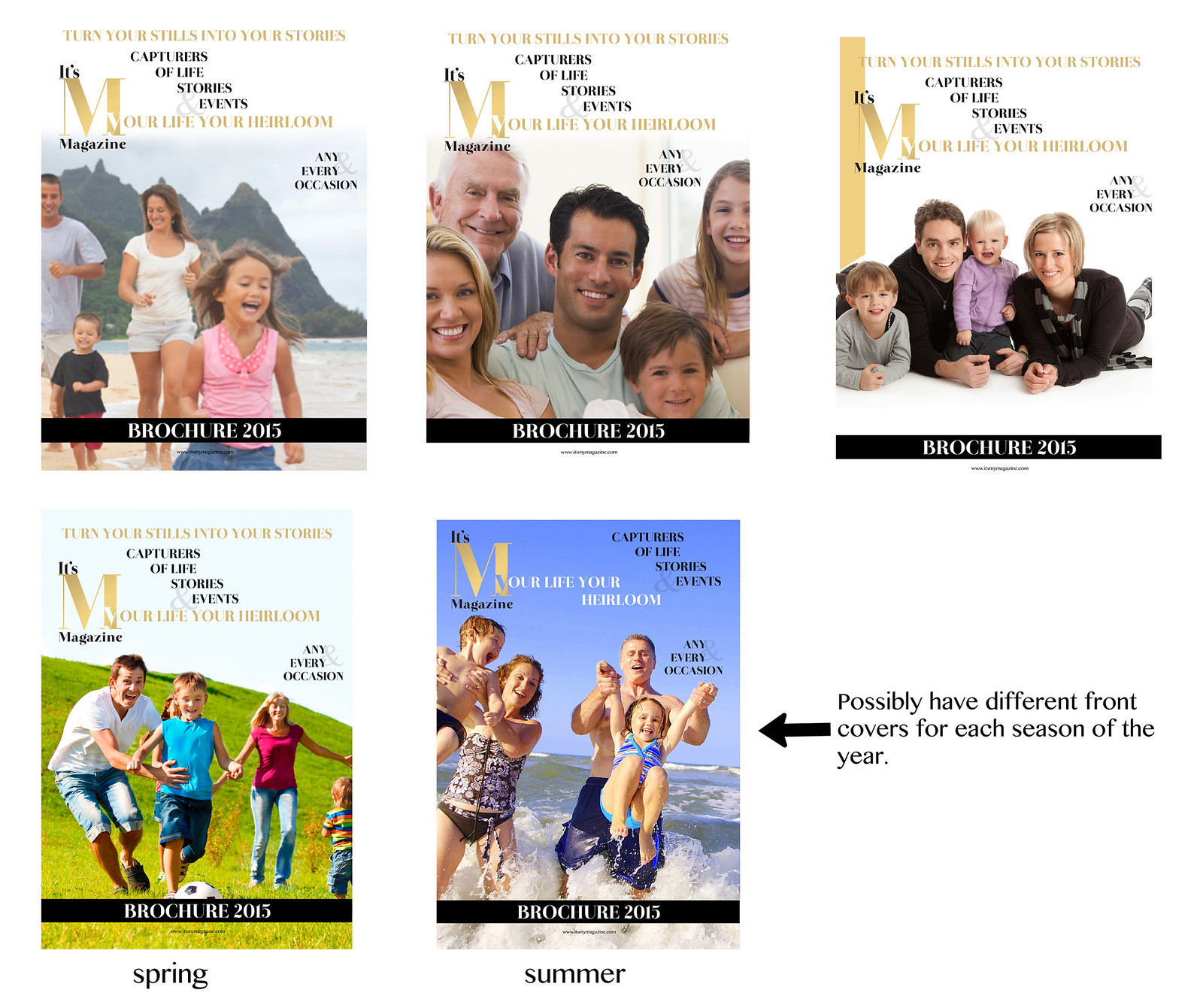The image showcases a collection of five "It's Your Life, Your Heirloom" magazine covers, each bearing the slogan "Turn your stills into your stories: Captures of life stories and events." These appear to be customizable brochures where families can feature their own photographs. Arranged in two rows, the top row has three covers while the bottom row has two. 

The first brochure, dated 2013, depicts a family of four—a man, a woman, a boy, and a girl—running on a beach with mountains in the background. The second cover also from 2013, shows the same family now joined by an older gentleman, possibly indicating the inclusion of grandparents. The third image, another 2013 cover, features a man, a woman, and two young children laying down outdoors. 

In the bottom row, the fourth cover shows a family with three children running on a grassy hill, again featuring the same caption at the top. The fifth brochure, marked summer 2015, is set against a blue sky and ocean backdrop, showcasing a man and a woman in swimsuits playfully swinging their young children into the waves. This particular cover also prominently displays the word "Summer."

The images seem brand new and the different families featured consist primarily of parents and children under the age of five. This collection is likely part of an advertisement, possibly highlighting the magazine's seasonal variety and customization options.